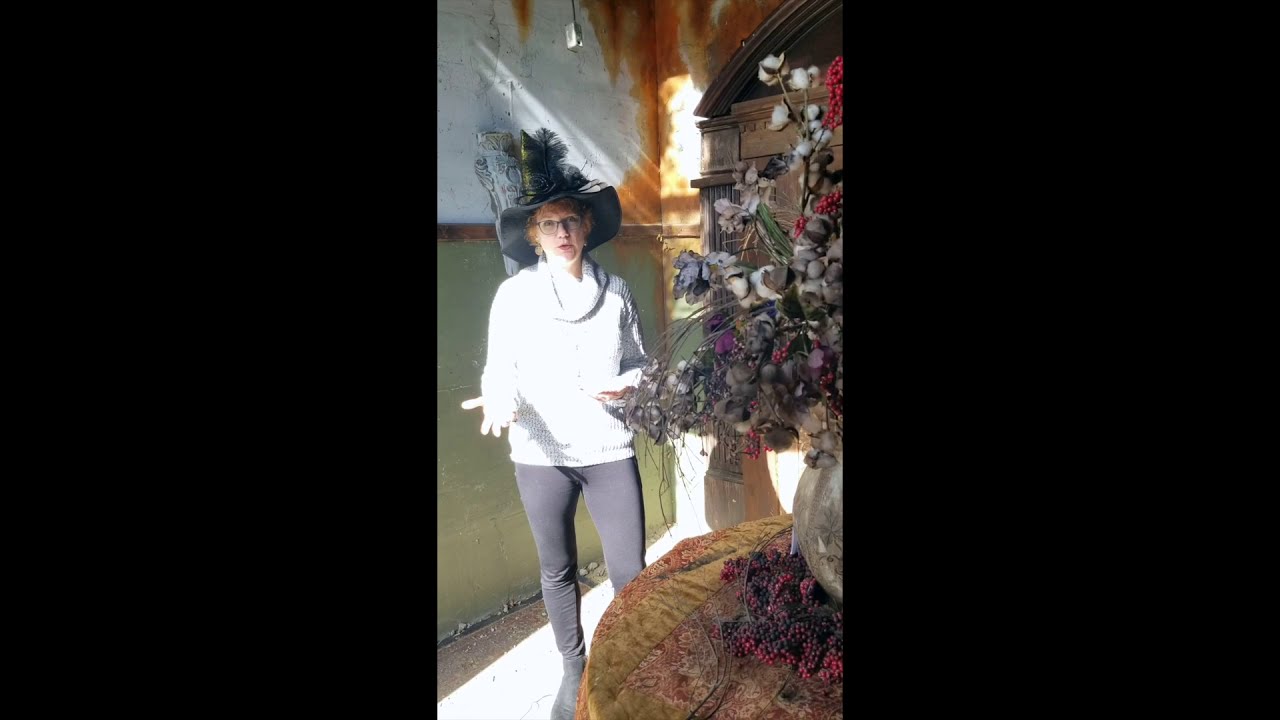The image features an older woman with short red hair and glasses, standing indoors next to a round wooden table adorned with a large vase of colorful flowers, some of which may include blue and green blooms, and possibly even wilted or dark flowers. She is dressed in a white turtleneck sweater, black leggings, and black ankle boots. On her head, she wears a distinctive, elaborate black witch's hat adorned with black feathers, resembling a fancy or bonnet-like hat. Her right hand is extended outward, and her mouth is partially open, suggesting she is mid-sentence, possibly explaining something. The background includes a partially rusted or water-damaged wall, with the upper portion painted white and the lower section green. Natural sunlight illuminates the scene, indicating it is daytime, and a heavy wooden doorway adds to the rustic ambiance.